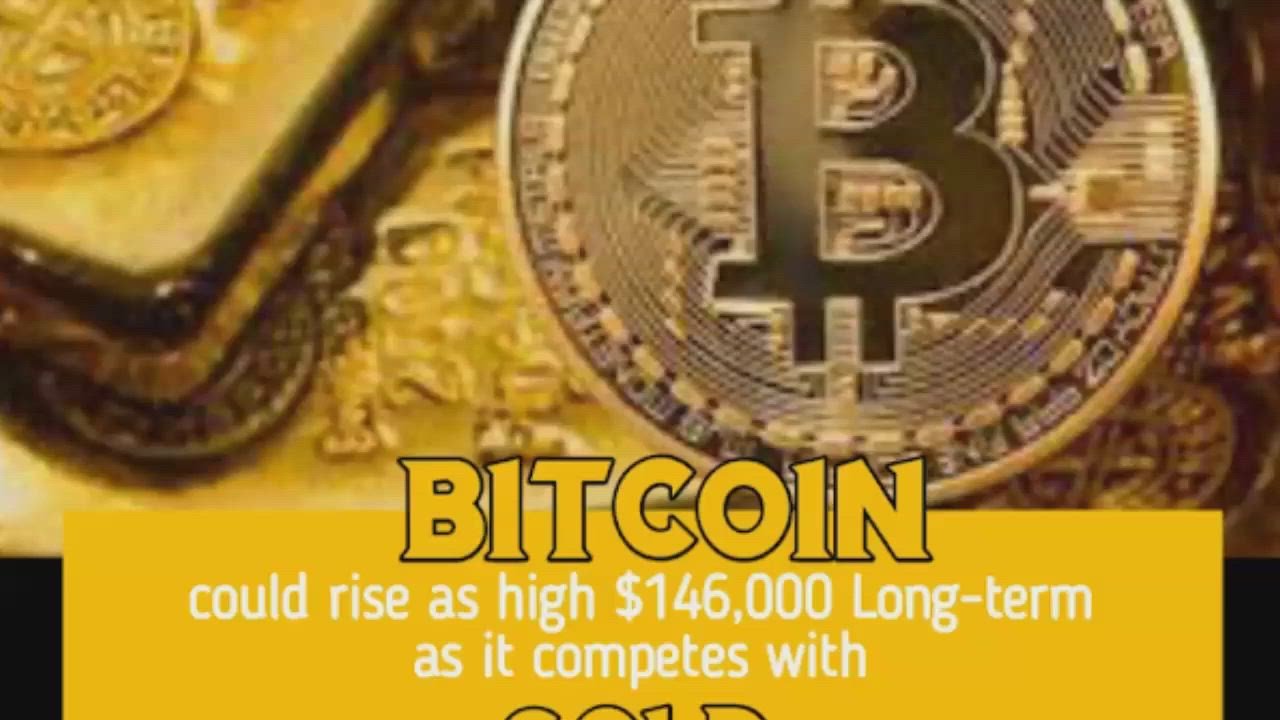This is a detailed Bitcoin advertisement with a predominantly yellow and gold background, accentuated by a black section filling the lower left quarter and a thin black border along the bottom right edge. Central to the image is a prominent, round coin featuring the iconic Bitcoin "B" symbol. Below this coin, the word "Bitcoin" is boldly displayed in yellow text with a black outline. Underneath the word "Bitcoin," the advertisement claims that Bitcoin could rise as high as $146,000 long-term as it competes with gold. Although the word "gold" is partially visible, only the top edges of the letters are discernible, cut off by the frame of the image. A golden bar is positioned in the upper left corner, while another circular Bitcoin image, partially cut off at the top, occupies the upper right corner. The ad aesthetically merges elements of both Bitcoin and gold, symbolizing the emerging competition between the two assets in wealth investment.